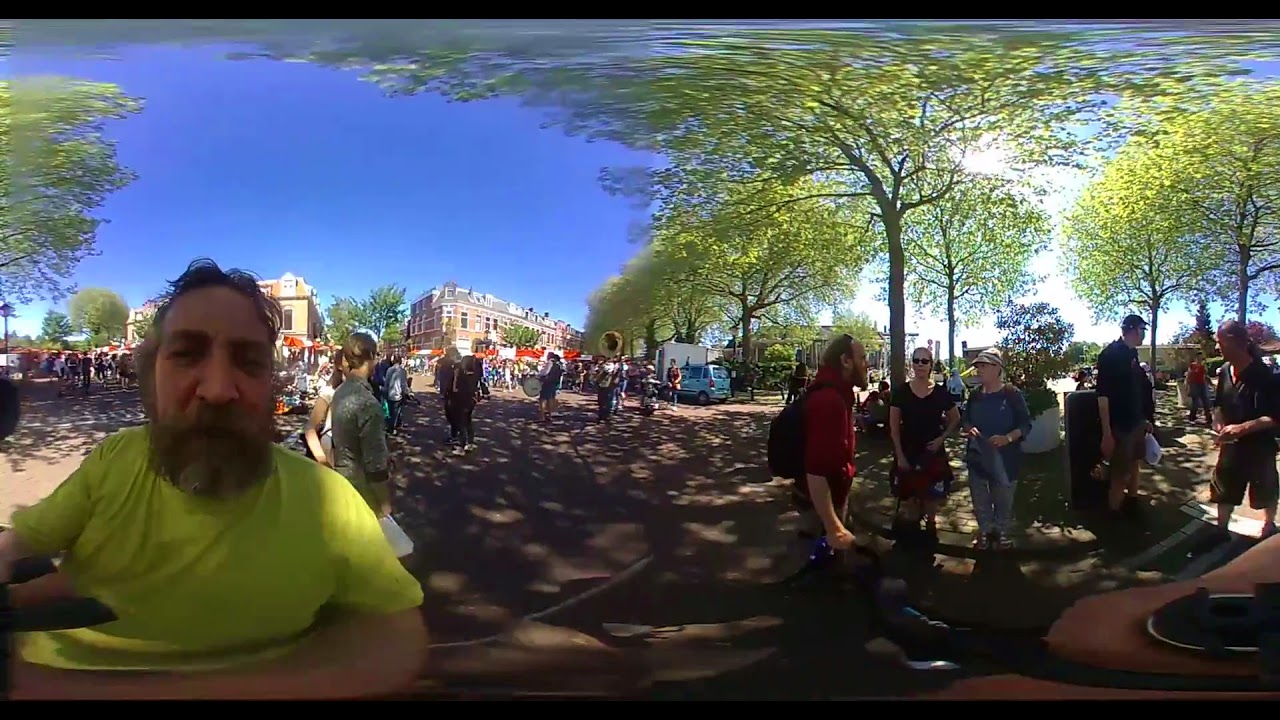The photograph is rectangular with solid black bars framing the top and bottom, giving it a panoramic feel that slightly distorts and rounds the image. The scene captures a bustling outdoor festival set in a park-like, open area with patio stones and a road. The setting features many large, tall, neatly manicured trees with bright green leaves, and a vibrant blue sky with a few scattered white fluffy clouds.

Prominently in the foreground on the left side, a white man with a beard and salt-and-pepper hair sits facing the camera, wearing a lime-colored, or fluorescent yellow, t-shirt. His appearance is casual, with uncombed hair and a relaxed demeanor. Behind him, the festival unfolds with groups of people scattered throughout the area. 

On the right side, a band is visible, featuring a musician with a tuba and another with drums, indicating live music. Nearby, a bearded man in a red shirt and backpack converses with two women wearing sunglasses.

The background is lively, showcasing more people walking or standing on the concrete ground. Overhead, there are red and white canopy coverings, likely shelters for vendors. The background also features tall brown buildings that may be apartments, nestled among additional trees, enhancing the sense of a vibrant community event under a beautiful sunny sky.